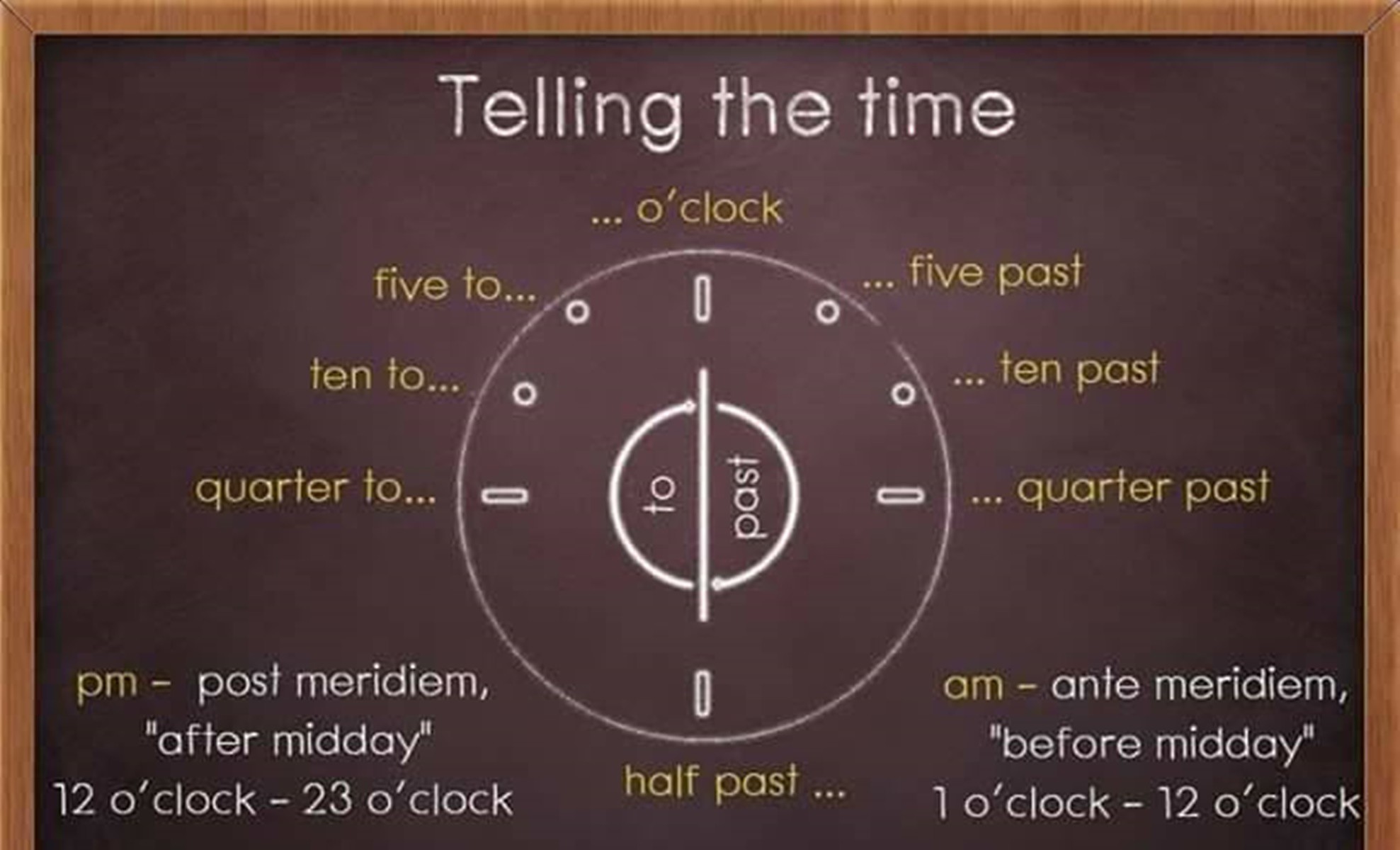This image is a framed informational poster designed to explain how to tell time on an analog clock. The frame is a simple, medium brown wood that encloses a dark brown horizontal poster. At the top center of the poster, in large white letters, it reads "Telling the Time."

Below the title is a white circle representing a clock face, displaying prominent vertical and horizontal dashes at the 12, 3, 6, and 9 o'clock positions. Smaller circles are positioned near the 1 and 2, and the 10 and 11 o'clock marks. A white line runs vertically through the circle, and surrounding it are circular arrows indicating a clockwise pattern. In the semicircle to the left it reads "to" in white, and in the semicircle to the right it reads "past." 

The clock is segmented into distinct time intervals labeled with terms such as "o'clock" at the top, "5 past," "10 past," "quarter past," "half past," "quarter to," "10 to," and "5 to," effectively guiding the reader in both directions around the clock.

At the bottom, the poster provides definitions for AM and PM. On the left, it explains "PM" (Post Meridiem), which means after midday, from 12 o'clock to 23 o'clock. On the right, it explains "AM" (Ante Meridiem), which means before midday, from 1 o'clock until 12 o'clock.

Overall, this neatly framed instructional poster serves as a comprehensive guide for understanding the positions and terms associated with reading an analog clock.